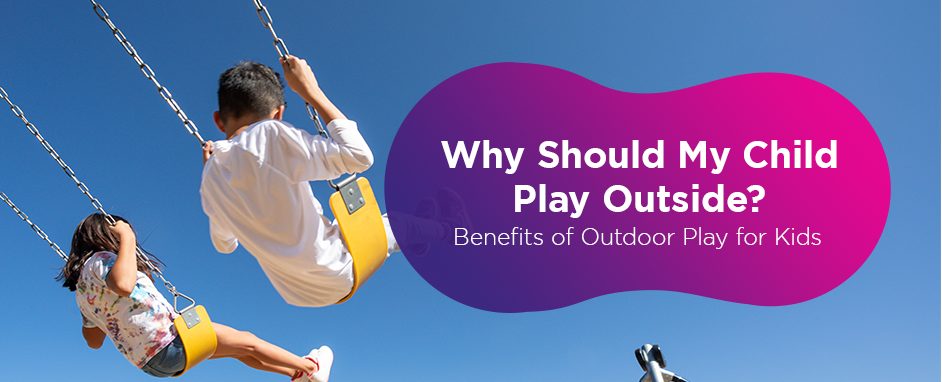The advertisement, set against a light blue sky-like background, focuses on the question, "Why should my child play outside? Benefits of outdoor play for kids," displayed in white text within a peanut-shaped gradient graphic that transitions from dark purple on the left to light pink on the right. Dominating the left side of the image are two children in mid-swing on yellow swings: a boy on the right and a girl on the left. Both children wear white shirts, with the girl's shirt featuring a colorful tie-dye pattern of blue, pink, and purple. They are also dressed in shorts and white shoes. The motion of swinging is emphasized by the visible arc of the swing chains stretching towards the top left corner of the image.